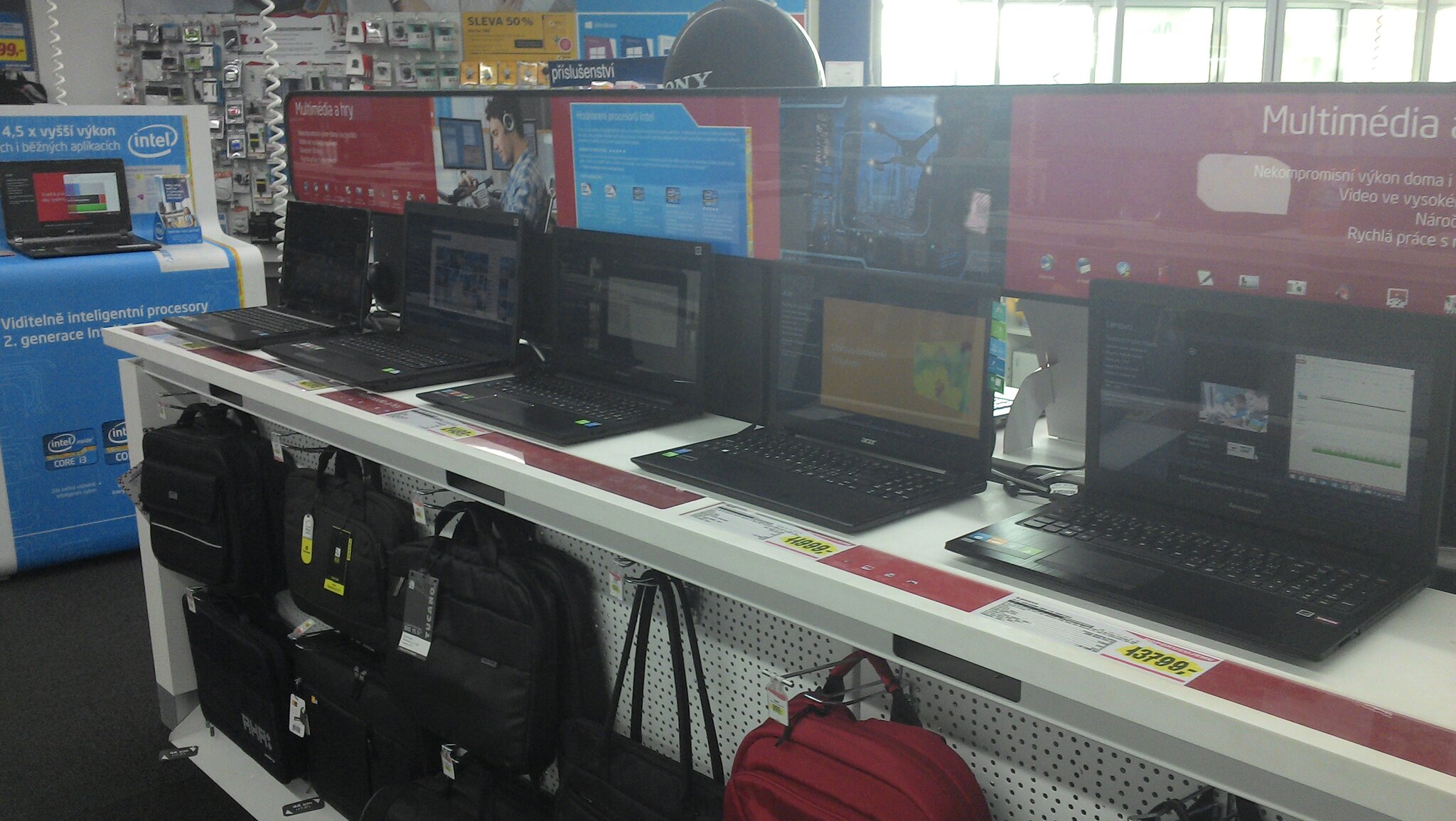This amateur photo, taken inside a brightly lit computer store, captures a row of laptops or Chromebooks lined up on a desk, their screens mostly on, with one exception where the screen appears to have gone dead. Below the laptops, a variety of laptop cases and bags are arrayed on hooks, predominantly black with various handle styles, and one red bag resembling a backpack. Price tags, some in yellow, and white specification lists are visible in front of each laptop. The image background features a large Intel advertisement and other signs, indicating this store might be in a Slavic-speaking region. Sunlight pours through open doors at the back of the store, casting a glow over the scene and enhancing the overall brightness despite the slight blurriness of the photo.